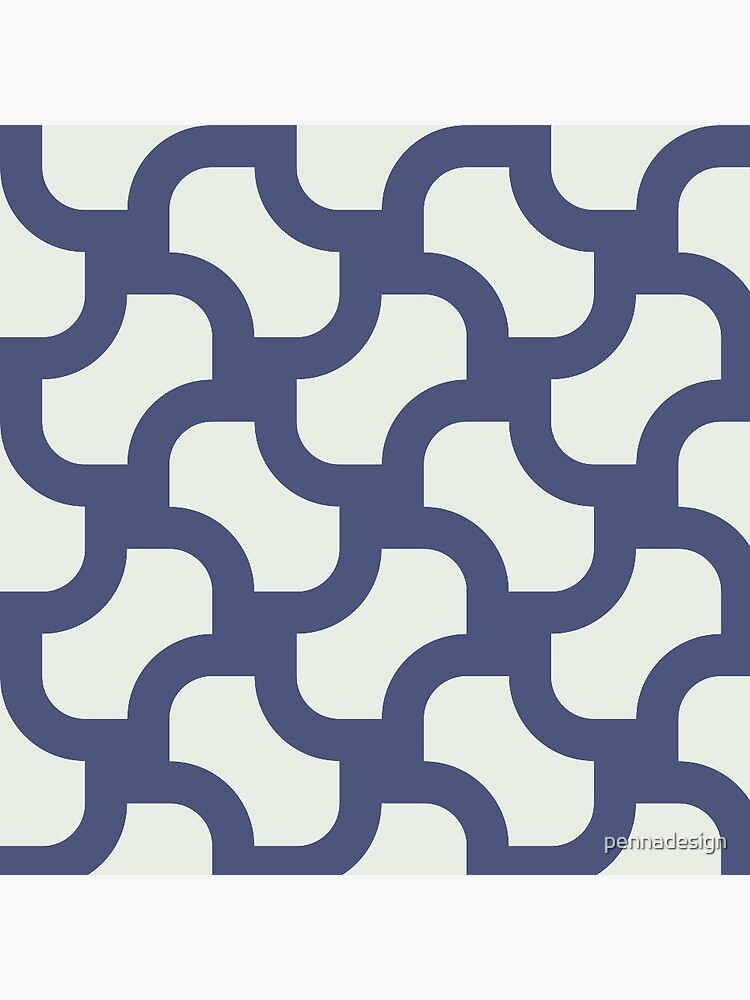The image features a digitally rendered pattern prominently displaying a design mimicking interlocking shapes reminiscent of a stretched figure eight or an apple core at various angles. This pattern covers the entire image, creating a detailed arrangement that evokes the look of chainmail or tile. The color scheme consists of dark cornflower blue shapes against a very light sky blue background, lending the design a clean yet intricate appearance. Adding to the composition's polished look is the "Pena Design" watermark located in the bottom right corner, indicating its creator. The overall pattern is symmetrical and continuous, bringing to mind samples of bathroom or floor tiles one might find in a home improvement store.